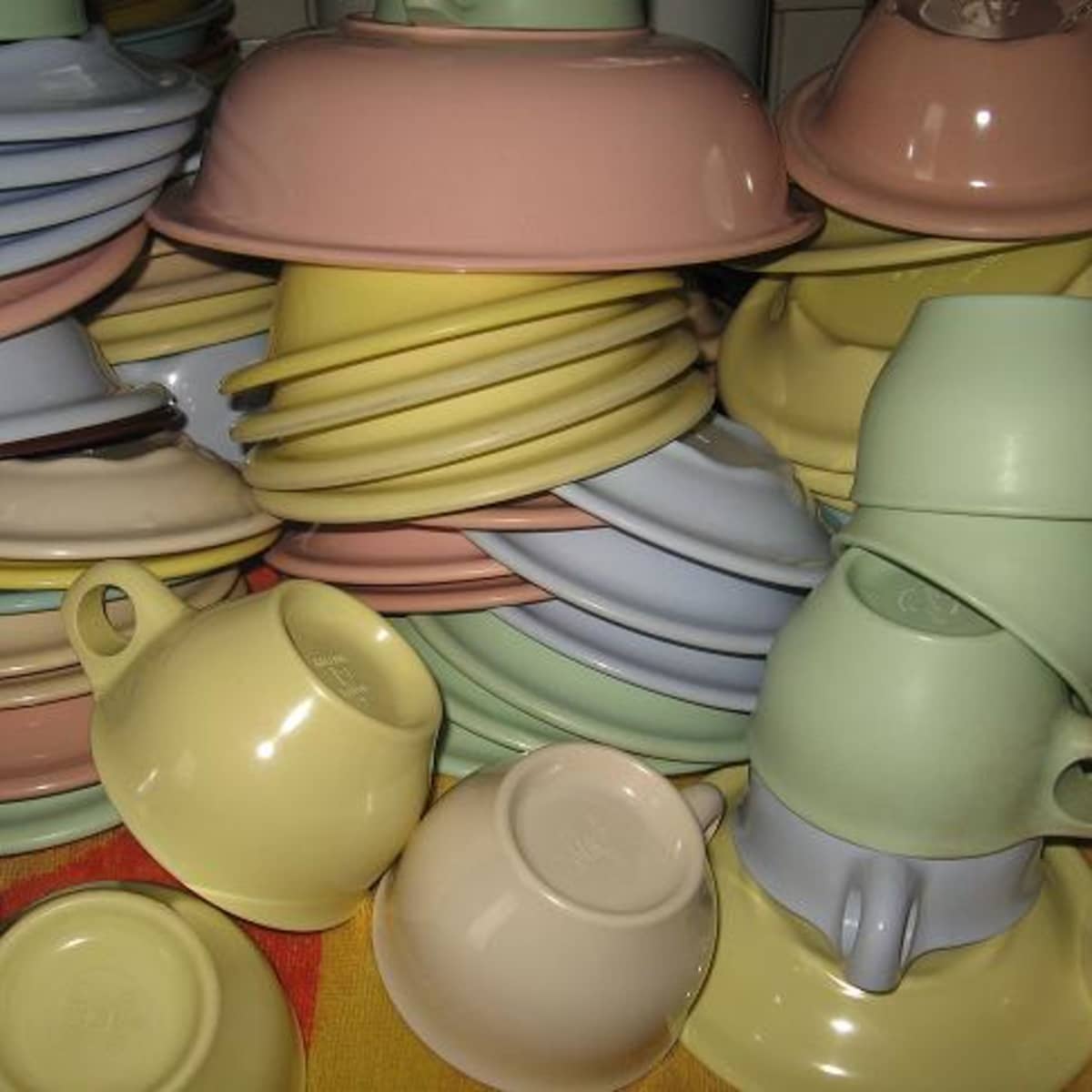The image showcases a vibrant and colorful collection of vintage melamine ware, reminiscent of mid-century restaurant dishware. The pieces—including bowls, plates, saucers, and coffee cups—are all stacked upside down, with the cups laying on their rims and their bases facing up. The dishware features a palette of pastel shades, including a dusty rose pink, light blue, harvest gold, tan, and a light sage green. The collection is presented in four distinct rows, creating a visually appealing arrangement. Most of the cups and mugs are positioned toward the front, with some grouped side by side and others stacked vertically. This assortment of thick, durable melmac pieces fills almost the entire image, all set against a yellow cloth adorned with red details, enhancing the overall aesthetic.